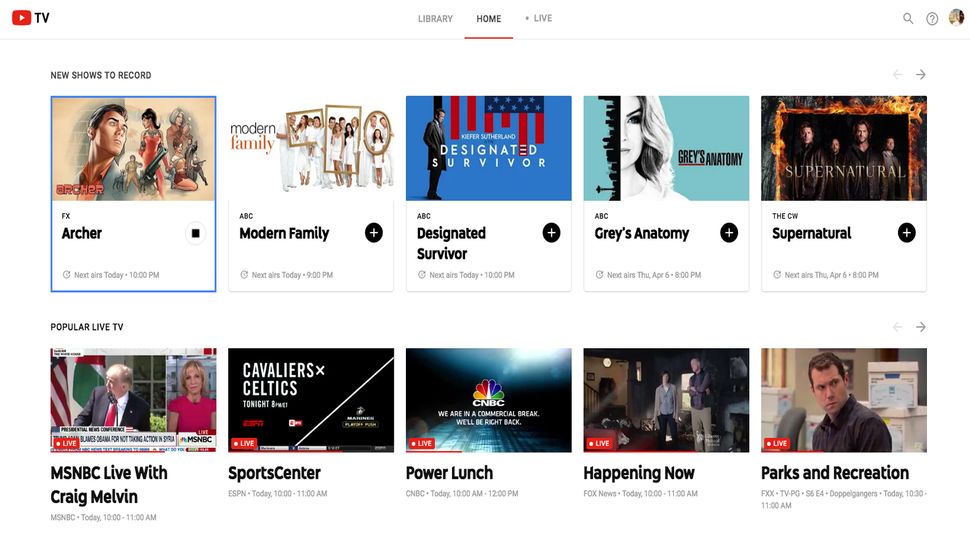This rectangular image, oriented with the longer side extending from left to right, appears to be a screenshot from YouTube TV. The predominant color in the background is white. At the top left corner, there is a red box featuring a white play button, signifying the YouTube logo. Adjacent to this logo is the word "TV."

Across the top center portion of the image, there are navigation options labeled "Library," "Home," and "Live." The "Home" button is currently selected, as indicated by its bold font and an underline. On the far right side of the top bar, there are three icons: a magnifying glass for searching, a question mark for assistance, and an account icon representing the user.

The main body of the image displays a selection of shows available for the user to watch. There are two horizontal rows, each containing five thumbnail images of different shows. In the top row from left to right, the shows featured are "Archer," "Modern Family," "Designated Survivor," "Grey's Anatomy," and "Supernatural." In the bottom row, the shows listed are "MSNBC Live," "Sports Center," "Power Lunch," "Happening Now," and "Parks and Recreation."